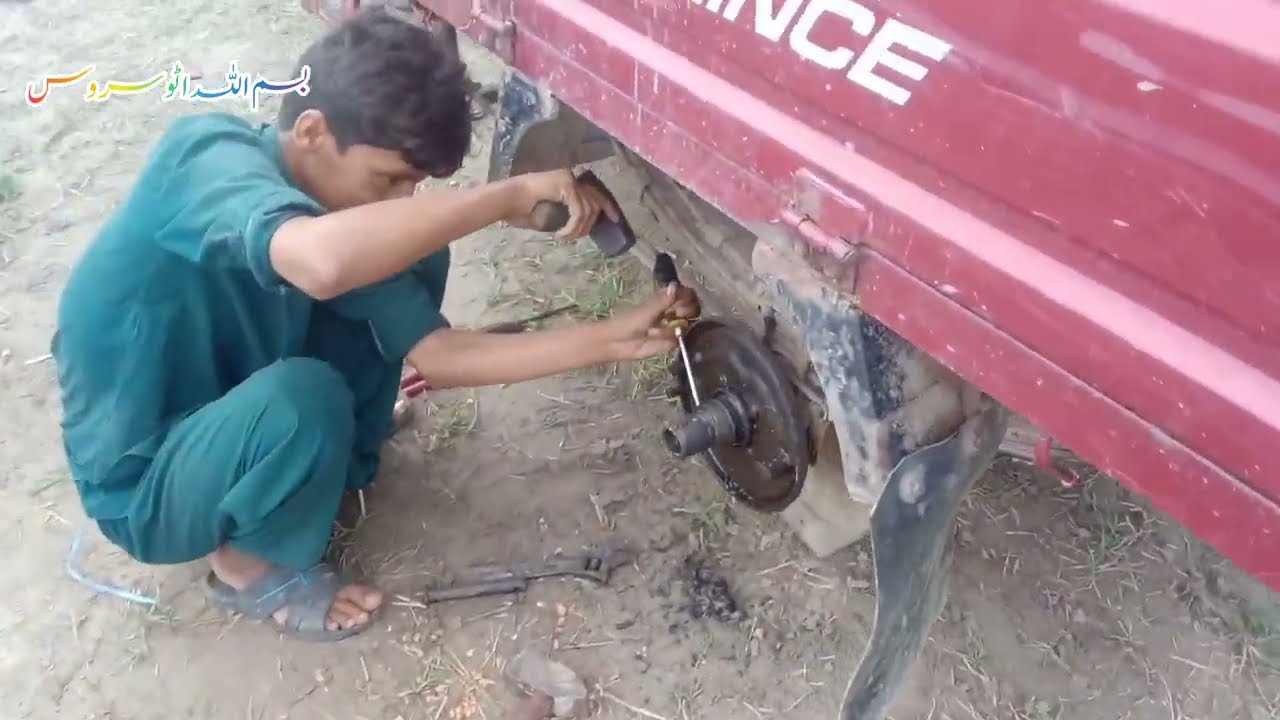In the photograph, a young boy with short, poofy brown hair and light brown skin is crouching on a dirt floor, attentively working on the wheel axle of a red vehicle, which is lifted up without its tire and rim. Positioned on the left side of the image, the boy is wearing an all-green outfit comprising a shirt and pants, resembling a mechanic’s uniform. His feet are clad in open-toed sandals. With a focused expression partially veiled by his arms, he firmly grips a small hammer in his right hand and a screwdriver in his left, appearing to tap the screwdriver with the hammer to possibly break or detach a rusted or seized component of the vehicle. Below him, a wrench lies on the dirt floor scattered with pieces of straw. A distinct oblique line in the composition marks the border between the dirt area and the side of the vehicle. In the upper left corner of the image, there is some Arabic writing in rainbow colors.